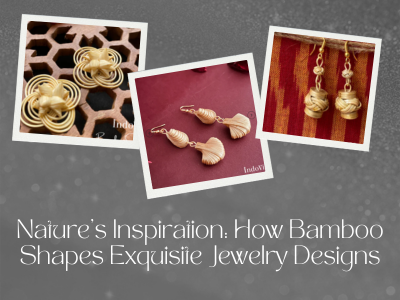This promotional graphic showcases exquisite jewelry designs inspired by bamboo, featuring a detailed collage of three different pieces of jewelry against distinct backdrops. The upper left photo presents a close-up of a golden brooch or pendant with intricate metalwork that replicates the segments and nodes of bamboo, set against a dark background with a hexagonal honeycomb pattern. The central image displays a pair of elegant earrings, resembling delicate bamboo shoots, resting on a rich burgundy background. The image on the right portrays another pair of cylindrical earrings that echo the bamboo motif, set against a light red and dark red striped background. The overall design is unified by a gray background adorned with faint white spots, and the tagline, “Nature’s Inspiration: How Bamboo Shapes Exquisite Jewelry Designs,” is prominently displayed, emphasizing the natural influence on these sophisticated pieces.